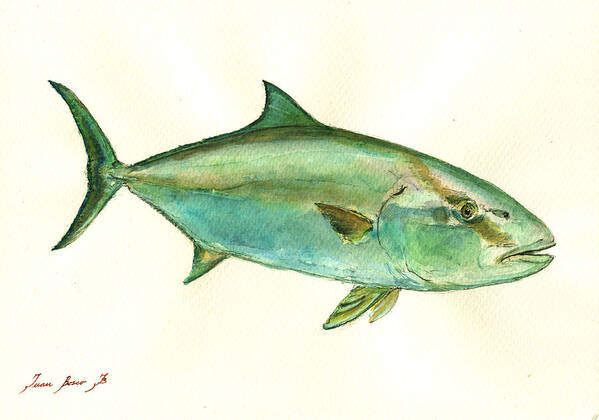The image is a detailed watercolor of a large fish, identified as a greater amberjack, facing to the left against a tan or cream-colored background. The fish exhibits a blend of bluish-gray and green hues, with additional colors ranging from dark green to lighter blue. Notable features include a distinctive brown stripe running from the top of its head, across its eye, and towards its mouth. The fish has two visible gills—one behind its head and another at the bottom—and two small fins, one positioned at the top and one at the bottom. The tail fin has a boomerang shape, colored in dark hunter green. The eye on the right-hand side of the fish is brown. The watercolor sketch, which resembles a greeting card, includes fine lines that add to the fish's texture. The artwork, signed by Juan Bosco in the lower left-hand corner, encapsulates the detailed and colorful depiction of the fish.